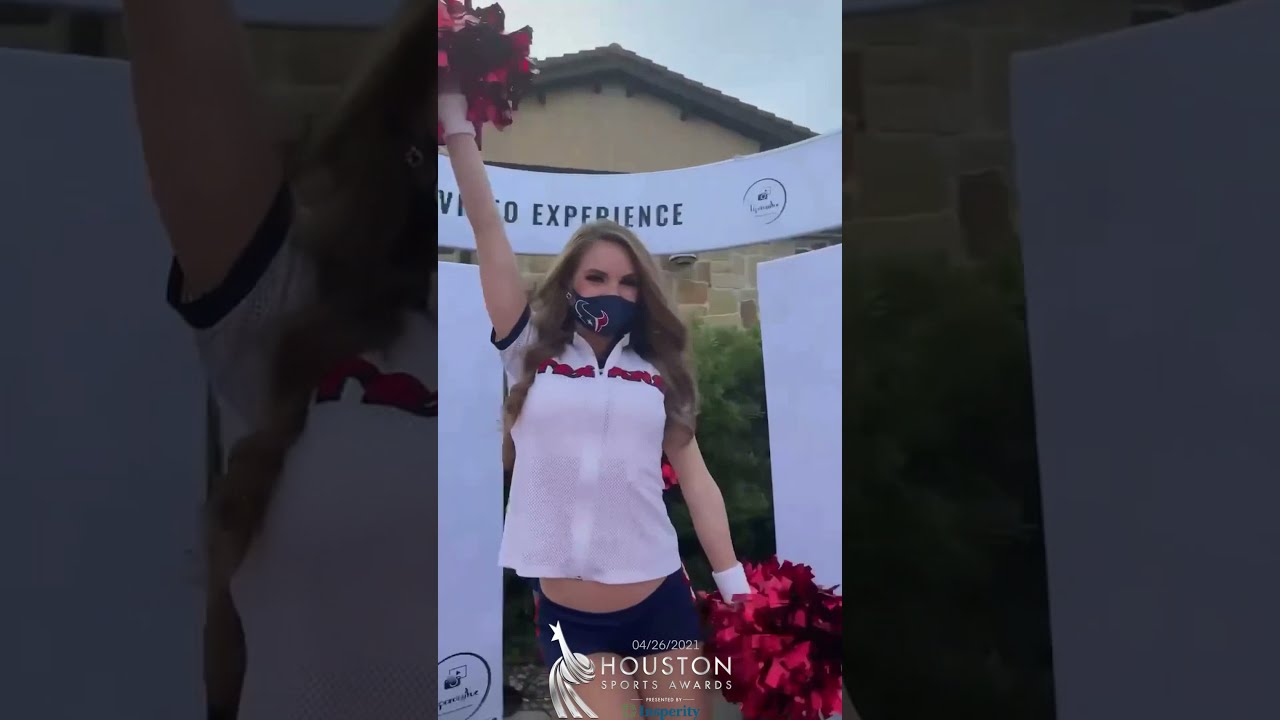The image features a blonde, white cheerleader posing in an alluring, cheerleading stance, with one hand up and one hand down, while holding red and black pom-poms. She’s wearing a face mask with a Houston Texans logo on it, positioned on the lower left corner. Her outfit consists of a collared, short-sleeve, white button-up top that exposes a bit of her midriff, paired with blue denim shorts. The backdrop includes a building and some greenery, with a banner that reads "Video Experience" and another text overlay at the bottom that says "Houston Sports Awards" dated 04-26-21. The scene also features white pillars on either side, fragmented side images, and various colors like navy blue, white, red, green, brown, black, and gray.